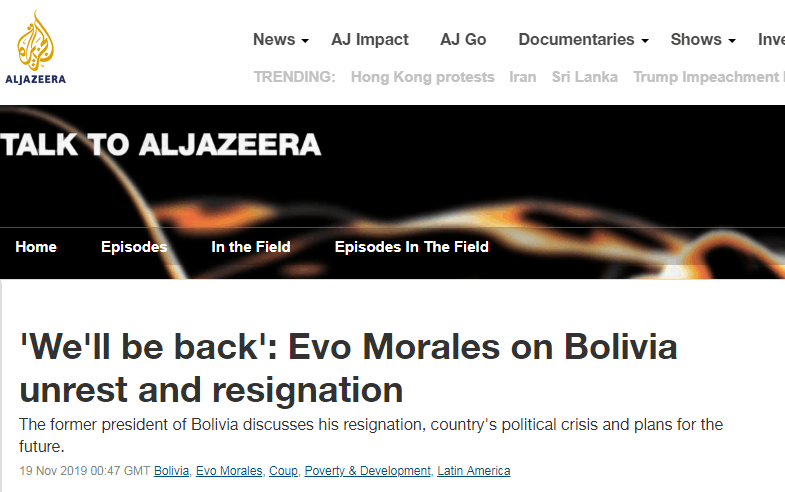This is a detailed screenshot of the Al Jazeera website homepage. In the upper left-hand corner, the name "Al Jazeera" is prominently displayed alongside its iconic logo, resembling a stylized drop of ink or flame. To the right, a navigation menu features tabs for various sections of the website, including "News," "AJ Impact," "AJ Go," "Documentaries," and "Shows."

Beneath the navigation menu is a prominent black bar with a flame design running through it, reading "Talk to Al Jazeera." This appears to be an advertisement for a program on the Al Jazeera network called "Talk to Al Jazeera." The title of the current episode featured is "We'll Be Back: Evo Morales on Bolivia unrest and resignation," indicating an in-depth interview or discussion with Evo Morales about the political turmoil and his resignation in Bolivia.